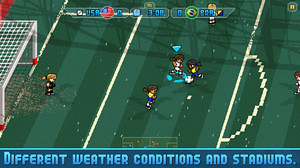This image is a detailed pixel art representation of a soccer game from a mobile video game, possibly advertised for iPhone or Android. The setting showcases different weather conditions in various stadiums, highlighted by blue text at the bottom. The left side of the field features a large white soccer net guarded by a goalie. On the field, there are three female players: one blonde with a ponytail in black, another with brown hair in a white outfit with a blue triangle above her, indicating that she is controlled by the player, and a third in a yellow shirt and blue pants, seemingly attempting to steal the ball. The scoreboard at the top indicates a match between the USA and Brazil, with scores and national flags visible. The overall scene captures an active moment during the game, emphasizing the interactive elements and vivid visual details.